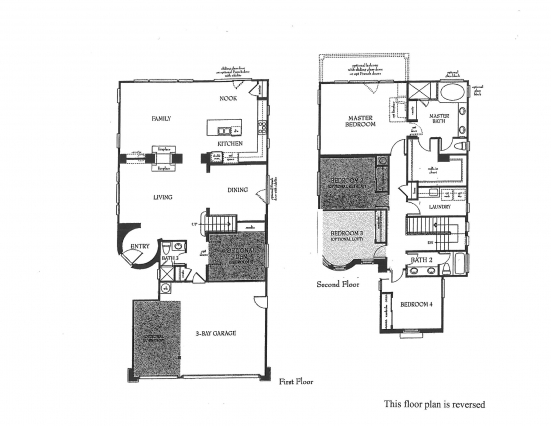Here is a detailed and cleaned-up caption for the described image:

---

The image displays detailed floor plans for a two-story house. The floor plan on the left side represents the first floor. At the front, there is a spacious three-bay garage. Adjacent to the garage is the main entryway, leading into a small hallway. On the left side of the hallway is a bathroom, while the right side features an open area allowing visibility to the upper floor. Moving further into the house, you enter the living room, which transitions into the dining area. At the rear of the first floor is a cozy family room, with the kitchen and breakfast nook situated to its left.

The floor plan on the right side of the image illustrates the second floor. On the left side, you will find Bedroom 3, and at the front right of the floor is Bedroom 4. Following these rooms are a shared bathroom and a stairway leading to the lower level. The layout also includes a laundry area. Notably, there is a dark open area on the left, which appears to be a balcony. Towards the back of the second floor, you will find the master bedroom, with the master bathroom conveniently located to its right.